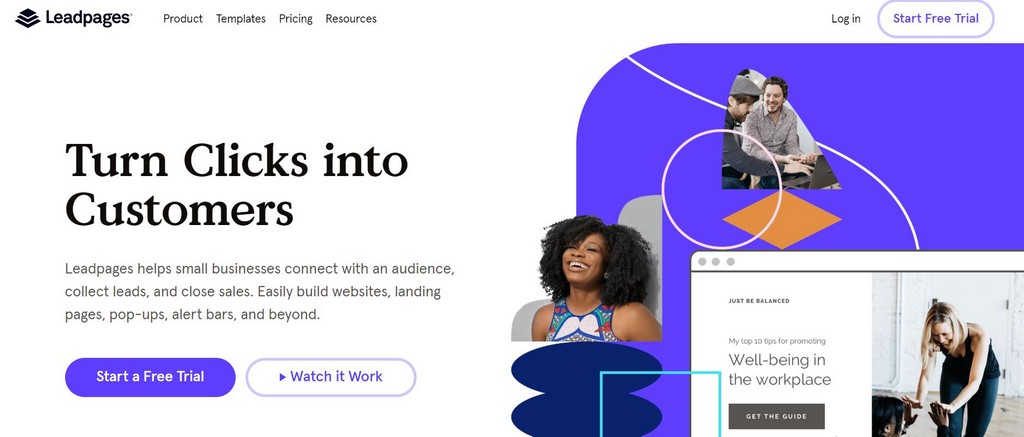The image, sourced from the Lead Pages website, showcases their homepage interface. Dominating the visual is a graphic depicting black pages that are large at the bottom and progressively smaller towards the top, symbolizing growth and hierarchy. To the left of this icon, the logo "Lead Pages" is prominently displayed.

Across the top of the webpage, the navigation bar includes options such as "Product," "Templates," "Pricing," and "Resources." Towards the far-right end of the navigation bar, there is a "Log In" option and a prominently featured circular button with a purplish hue that invites users to "Start Free Trial."

Central to the page, in bold black letters, is the headline "Turn Clicks into Customers." Below it, additional text explains that "Lead Pages helps small businesses connect with an audience, collect leads, and close sales. Easily build websites, landing pages, pop-ups, alert bars, and beyond."

Two call-to-action buttons are prominently displayed: a purple one labeled "Start a Free Trial" and a white one with an arrow labeled "Watch It Work."

Accompanying the text, on the right side of the image, are photos of individuals: an African-American woman smiling and looking upwards, a presumed yoga instructor high-fiving someone nearby, and two men engaged in conversation.